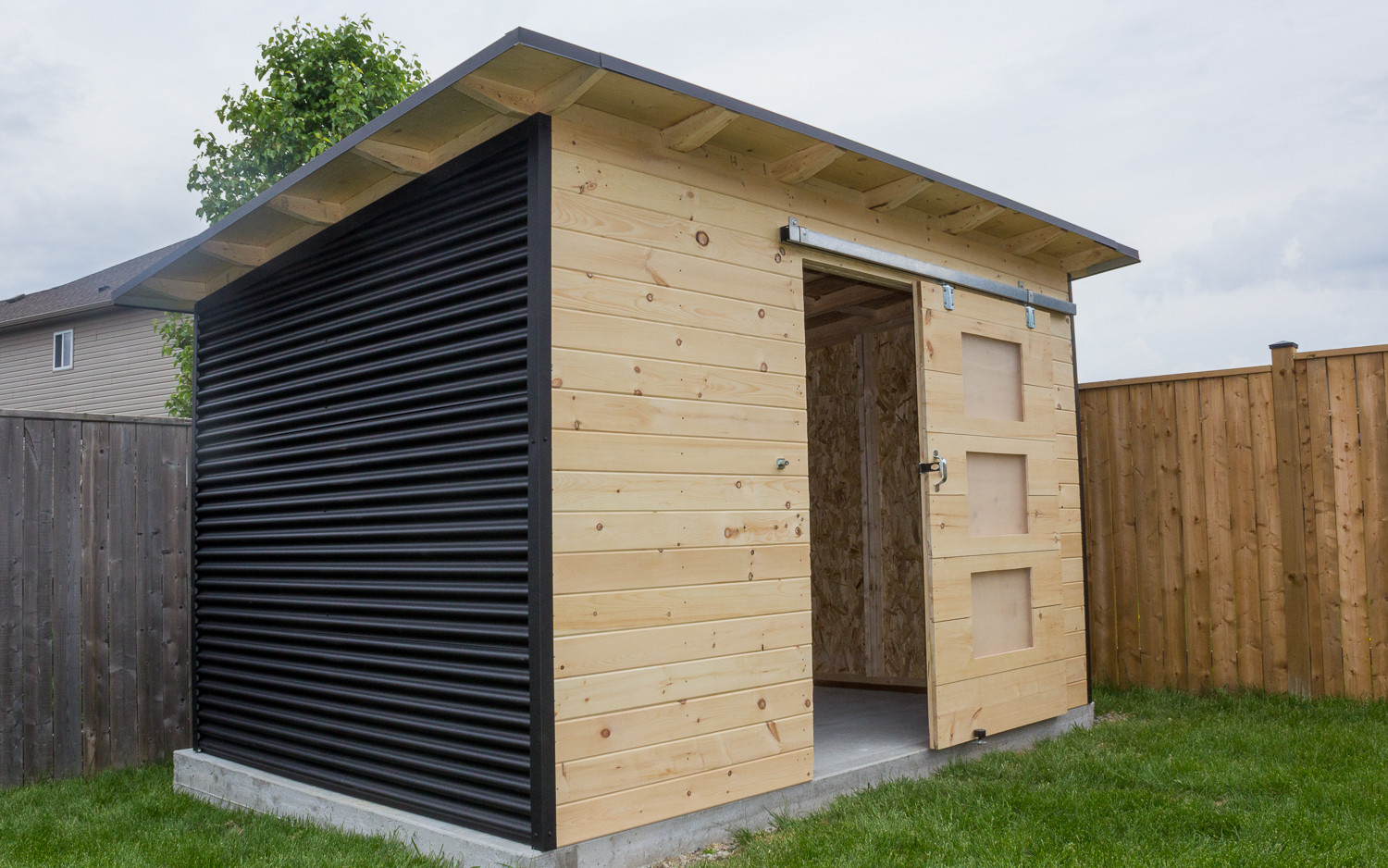This image depicts a newly built shed situated in a backyard, surrounded by a grassy area and enclosed by a wooden fence that stands just above head level. The shed is raised slightly on a gray concrete slab, giving it a sturdy foundation. The front of the shed is constructed from pale, likely varnished, pine boards, and features a sliding barn-style door on a rail that is currently partially open, revealing the unfinished interior. This door has three square cutouts arranged vertically in the center. Adjacent to the wooden front, the left side of the shed is covered in horizontally corrugated metal siding, reminiscent of roofing materials. The shed sports a flat roof that extends about a foot from the walls, with a slight slope from front to back to facilitate rain runoff and an overcast, gray sky above. Behind and to the right of the shed stands a wooden fence, and looming above this fence is a large tree. In the background, a separate house with a tan exterior and brown roof is visible, further emphasizing the backyard setting.